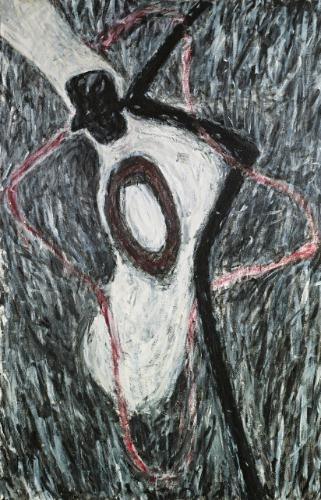The image portrays an abstract drawing with a densely scratched black crayon background, consisting of vertical streaks across a piece of paper. Dominating the image is a white, foot-shaped figure that extends from the upper left corner and tapers down to the center. This white shape contains an outline of a black, featureless face donning a top hat. The hat and face are solid black, resembling a crude mask or silhouette. The centerpiece of the foot-like shape includes a red circular or rectangular mark, adding to the intricate symbolism.

Bordering the white figure is a bold black line that begins at the top, winding its way down and bending at the ankle region before continuing to the bottom. Adjacent to this black line is a large circle, often perceived as a zero, positioned just forward of the ankle area. Encircling the entire artwork is a red and white cross-like symbol, wrapping beneath and emerging behind the image, suggesting a sense of confinement or frame.

In the overall abstract and chaotic composition, the white figure's outline vaguely implies arms holding a stick, giving it a character-like appearance. The black face and hat significantly contrast against the white body, which has been compared to a peanut shape. The background remains an intricate web of scribbles, enhancing the modern and enigmatic aura of the piece.